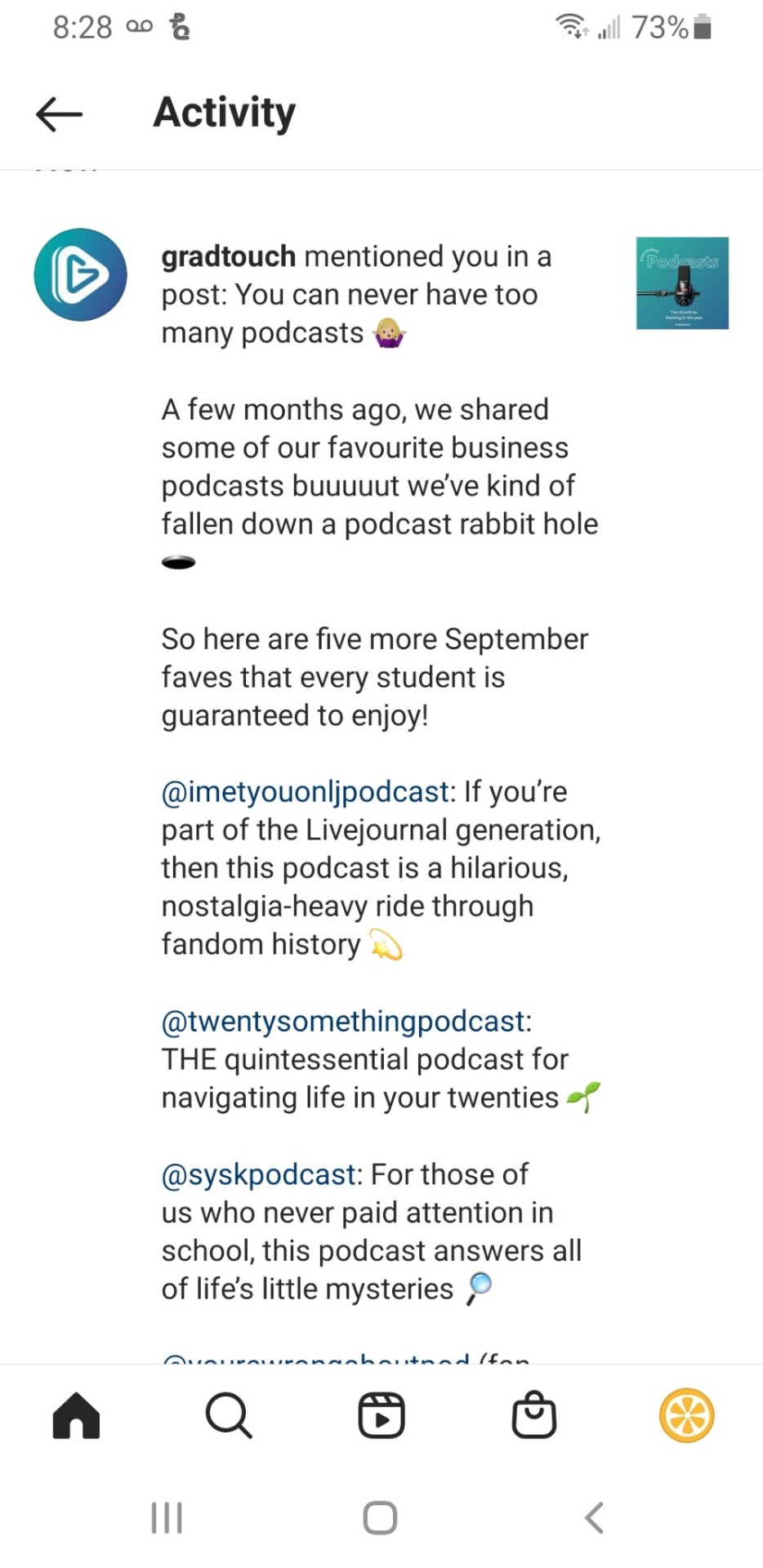**Caption:** 
The screenshot, taken from a mobile device, displays a time of 8:28 and a battery level at 73%. The screen shows an app or section entitled "Activity" where a user named "Brad Touch" has mentioned the viewer in a post. The content of the post praises the abundance of podcasts and shares a new list of favorite business podcasts for September. Highlighted recommendations include:

1. **Add I Met You on LJ Podcast** - A humorously nostalgic and fandom-centric podcast perfect for the LiveJournal generation.
2. **20 Something Podcast** - A go-to guide for navigating the complexities of life in your 20s.
3. **Sis K Podcast** - An informative podcast that answers intriguing questions for those who might have been less attentive in school.

The post tantalizingly continues with more content that is cut off at the bottom of the screen. The mobile device's navigation menu, including options such as Home and Search, is also visible at the bottom of the screenshot.